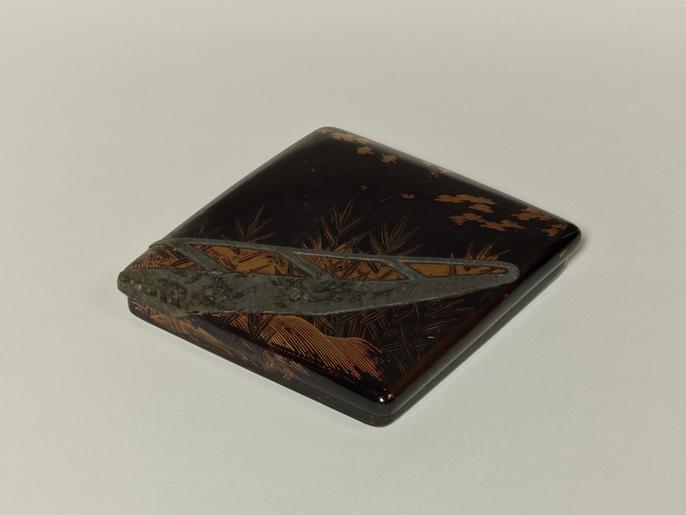The photograph depicts a small, shiny, and glossy black disc with intricate details. The disc features gold coloring, including gold leaves that elegantly emanate from its top part. There is also a distinctive silver piece jutting out from the bottom left corner, accented by gold elements embedded within it. The object is placed on a flat surface that appears to be either a beige table or a dull gray background, creating a modest contrast to the disc's opulence. The disc is turned at a slight angle, adding to its visual intrigue. While its exact nature is ambiguous, it resembles either an antiquated decorative coaster or an old, ornate watch with a vintage aesthetic.